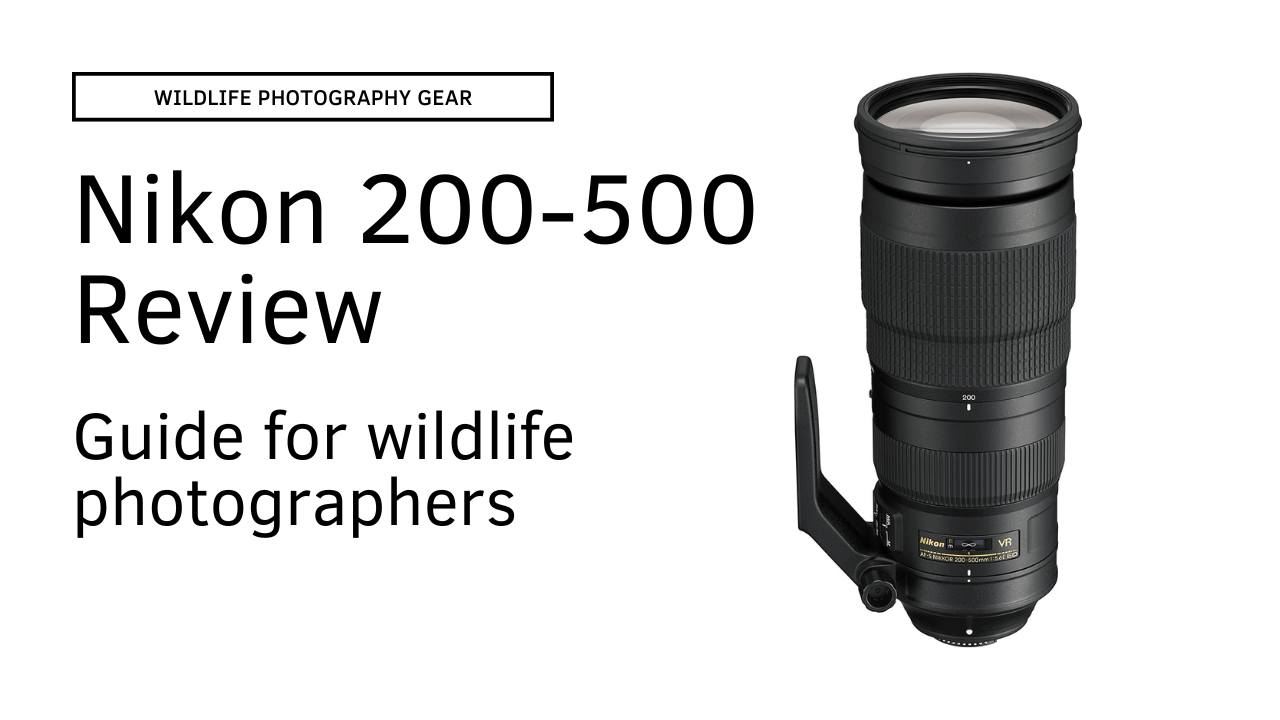The advertisement image showcases a detailed, professional photographic representation of a Nikon 200-500mm camera lens, specifically designed for wildlife photographers. The lens, entirely black with intricate ridges and a lever attachment on the left side, stands vertically against a white background, giving a floating impression. In the top left corner, there is a prominent horizontal rectangle with bold black text on a red and black background, stating "Wildlife Photography Gear." Beneath that, bold black text reads "Nikon 200-500 Review," followed by smaller text, "Guide for Wildlife Photographers." The overall composition merges realism in product depiction with clean, typographic graphic design elements.